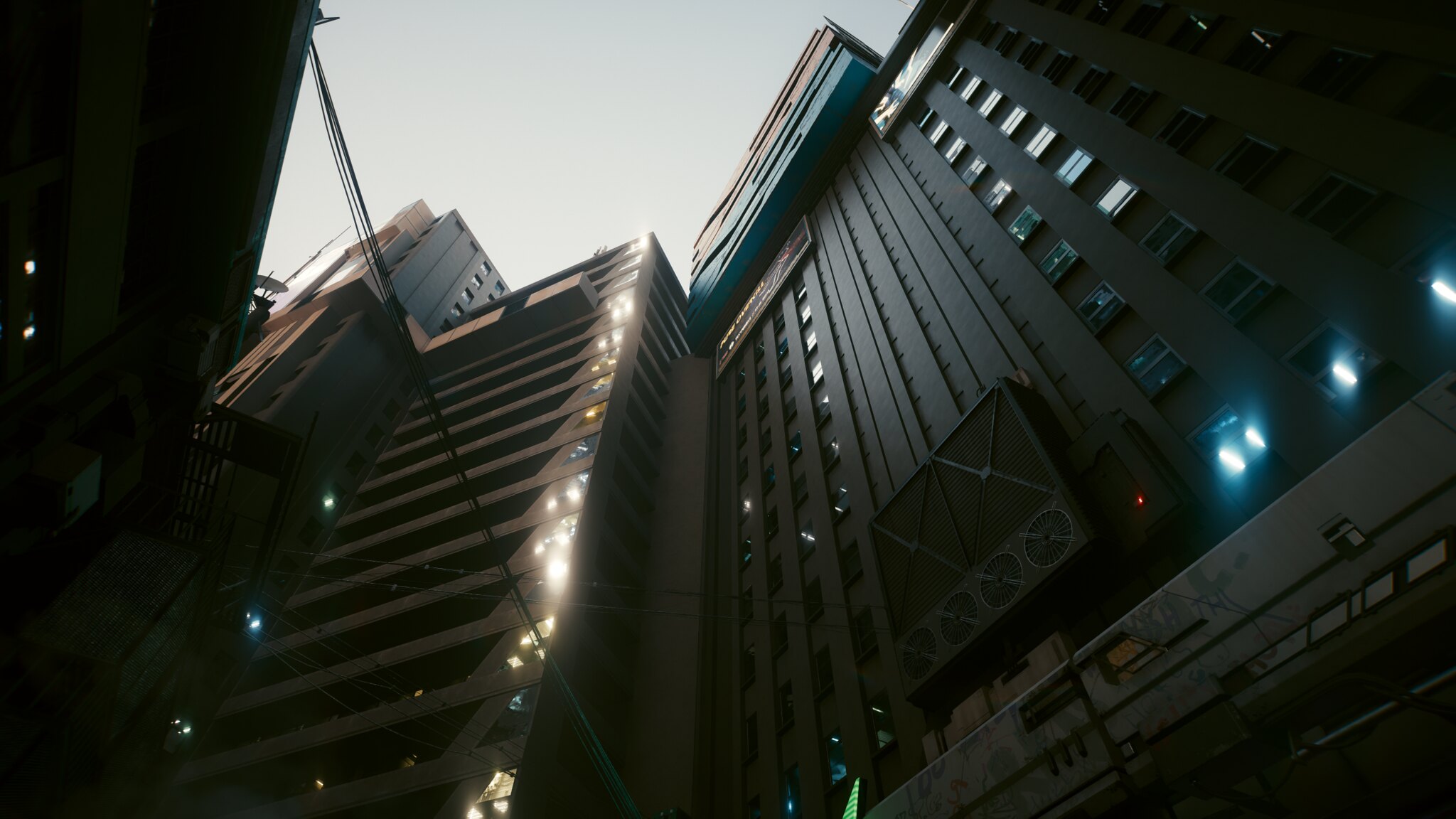An upward-view photograph captures a cluster of tall buildings from the perspective of someone standing on the street. The prominent building on the right, possibly AI-generated, features either a cement or brick facade. Attached to this building is a peculiar black structure, which might be a large speaker system or a ventilation unit. This apparatus consists of two rectangular speakers side by side, accompanied by a series of four round speakers.

The base of the building shows signs of ongoing construction, with scaffolding present. Rows of windows ascend up the sides of the building, some of which are emitting light, possibly indicating interior lighting from a parking garage or lighted stairwells. The top of the building has an additional blue and brown structure or level.

On either side of the building's upper sections, there are billboards. The lighting conditions create heavy shadows on the buildings, making it challenging to discern certain details. A power line extends across the left side of the image, adding to the urban atmosphere. 

In the background, to the left, another building with numerous windows is visible, featuring a satellite dish on its rooftop. The photograph is set against an overcast, gray sky, enhancing the subdued and moody tone of the scene. The left side of the image contains a dark, indistinct object that could be part of a building or another street element.